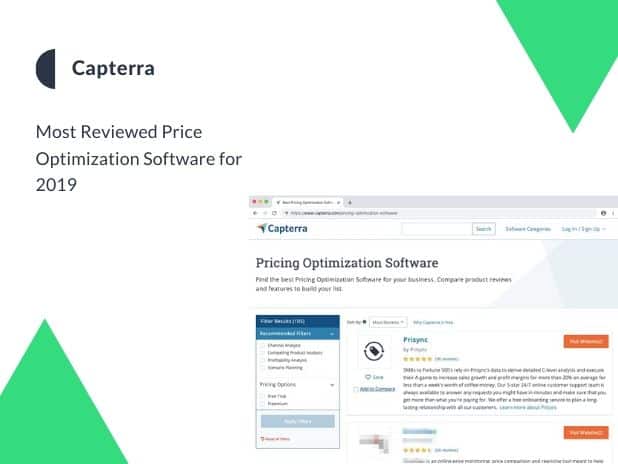This image showcases Capterra, the most reviewed price optimization software of 2019. Prominently, the name "Capterra" is displayed with a black semicircle alongside it. In the top right and bottom left corners, there are distinctive green shapes resembling partially cut-off triangles. A web browser screenshot occupies the lower right quadrant of the image, taking up about a quarter of the space. This screenshot features the Capterra website, with its name and colorful arrow-like logo at the top. Below it are typical web elements like search, sign-in, and sign-up options, followed by a section labeled "Pricing Optimization Software" with a brief description. Although the text is too small to read clearly, an EACA box with navy blue and lighter blue headings is visible, along with clickable options with orange bars.